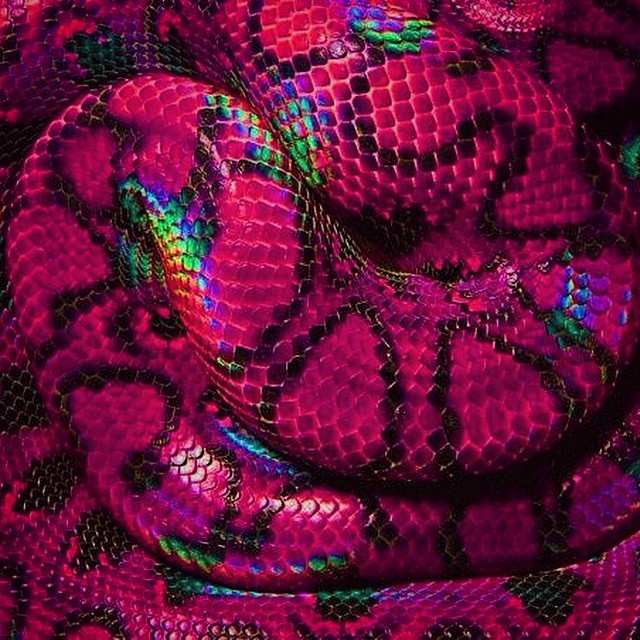This image is a highly detailed close-up of a snake's body, showcasing its intricate scales and vivid coloration. The snake is curled up, filling the entire frame with its textured surface. The overall appearance suggests that it's likely a computer-generated or heavily photoshopped representation rather than a real snake, given the extraordinary color palette. The scales exhibit a dominant magenta hue adorned with black stripes, while some scales reflect a holographic, iridescent quality, shifting through shades of blue, green, orange, and yellow under the light. The vibrant, almost neon rainbow colors create an eye-catching, surreal effect. There is no visible head, just the coiled, mesmerizing body, which intricately plays with light to produce this striking visual.